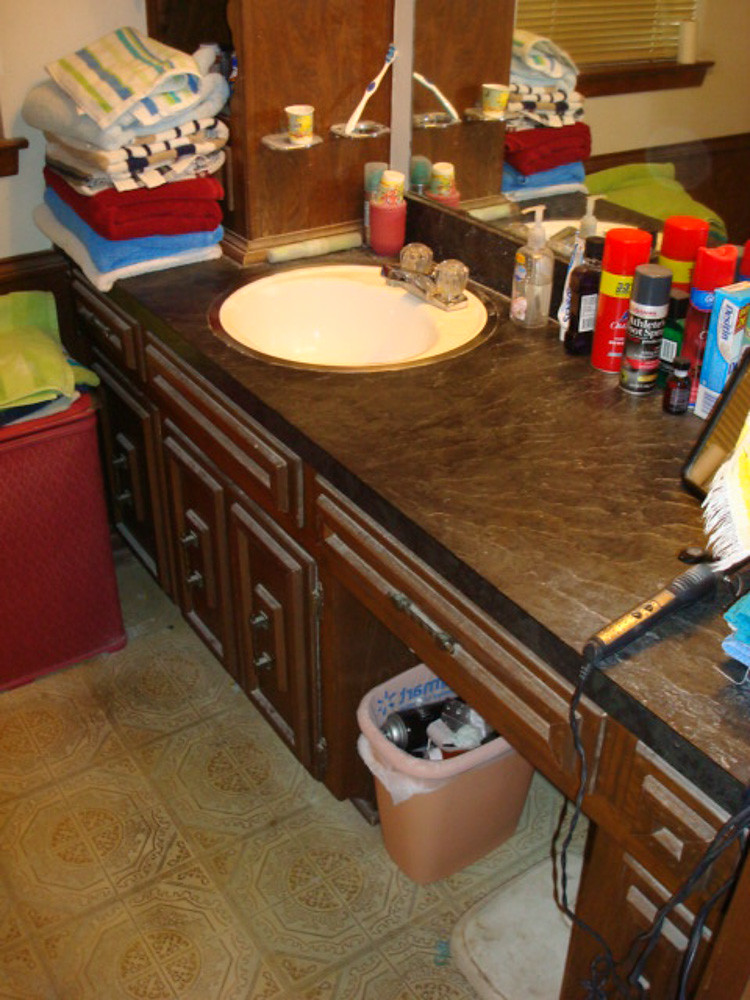This vividly colored photograph captures the interior of a bathroom centered on a dark wooden vanity. The vanity features multiple cabinets and a central space designed for seating. Below the vanity, a pale pink waste bucket is visible, filled with several empty bottles. The surface of the vanity is a dark brown laminate wood adorned with a variety of items.

To the left, there is a sink fitted with clear faucets. Piled up on the edge of the vanity are several folded towels in an array of colors: blue, red, brown, black and white, and white with green and blue stripes. Various bottles and cans are scattered across the vanity’s surface, including red and black cans of substances. A black curling iron with gold embellishments and visible buttons is also prominently displayed on the vanity.

At the back of the vanity, a mirror reflects the scene, including the towels and a window with drawn, tan shades. On the floor, a reddish square plastic case, possibly a laundry basket, contains more tiles, adding to the organized clutter of the bathroom.